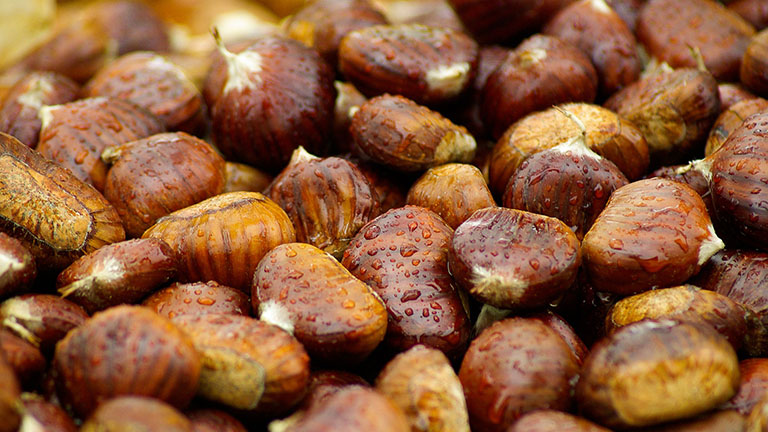The image is a highly detailed close-up of a collection of small, oval-shaped nuts, possibly macadamia nuts or hazelnuts, filling the entire frame. They range in color from dark brown to reddish brown to light brown, each having a distinctive white tip and a pointier end. The scene is captured with a tilted, diagonal top-down view, making it appear as though one is looking inside a can filled with these nuts. The nuts are covered with water droplets, suggesting they are fresh. The central focus of the image is sharp, while the edges, particularly the upper left corner, are blurry. A striped pattern runs longitudinally along the surface of each nut, adding to their textured appearance. The glistening droplets highlight the moisture and freshness of the nuts, enhancing the overall rich detail and depth of the image.